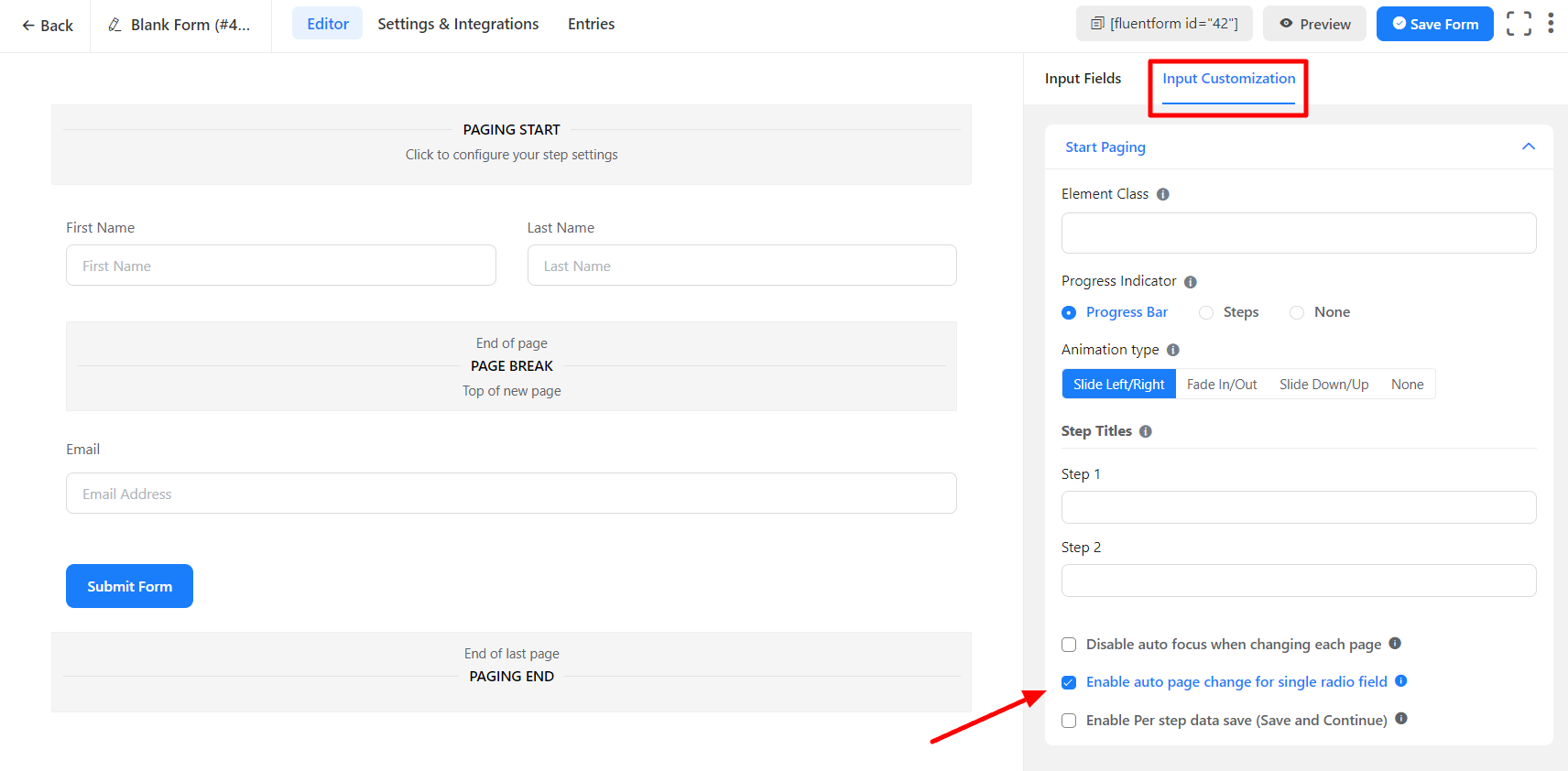The image displays a form editor interface. At the very top, there is a navigation bar featuring a back arrow labeled "Back", and icons for "Blank Form" with a pencil, "Editor", "Settings and Integrations", and "Entries". 

Beneath this, there is a configuration panel with the instruction "Paging start - click to configure your step settings." Fields for "First Name" and "Last Name" are present, followed by a page break labeled "End of page". 

The next section, marked as "Top of page", contains an "Email" field where users can input their email address. Below this, there is a "Submit Form" button, and another page break labeled "End of the page" and "Paging end".

On the right side of the screen, there is a sidebar. Here, details such as "Form ID", a "Preview" button, and a "Save Form" button are displayed. Additionally, there are sections for "Input Fields" and "Input Customizations", which is highlighted with a red rectangle.

Within the customization options, it says "Start Paging" with an upward arrow. Other elements listed include "Element Class", "Progress Indicator", and "Progress Bar" which has a dot next to it. The "Animation Type" options listed are "Side Left Right", "Fade In and Out", "Side Down", and "Up or None", with "Side Left Right" being selected. Below these, it displays steps "Step One" and "Step Two". There is also a checked option to "Enable Auto Page Change for Single Radio Field".